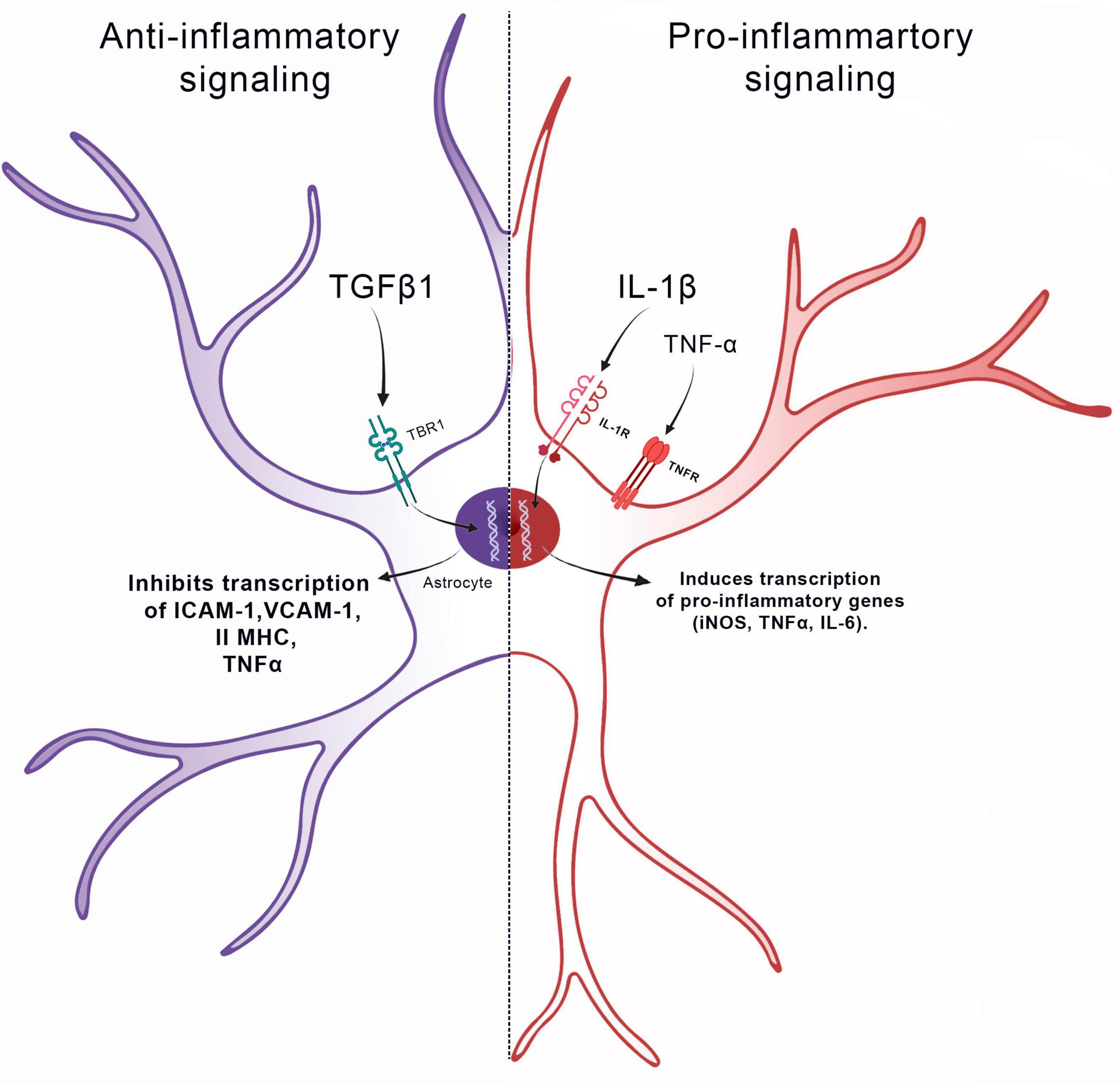The image is a detailed scientific diagram against a white background, depicting anti-inflammatory and pro-inflammatory signaling pathways in an astrocyte cell. The diagram is bisected by a dotted line, separating the left purple-hued half from the right red-hued half. The left side of the diagram is labeled "anti-inflammatory signaling" and includes the text TGFβ1 with an arrow pointing to the cell's center. It describes inhibiting transcription of ICAM-1, VCAM-1, 2MHC, and TNFα. The right side, labeled "pro-inflammatory signaling," displays the text IL-1β and TNFα, indicating the induction of transcription of pro-inflammatory genes such as iNOS, TNFα, and IL-6. Both halves show multiple extensions resembling nerve endings or cellular tendrils. The central oval shape is labeled “astrocyte,” with each half mirroring the respective signaling pathways.